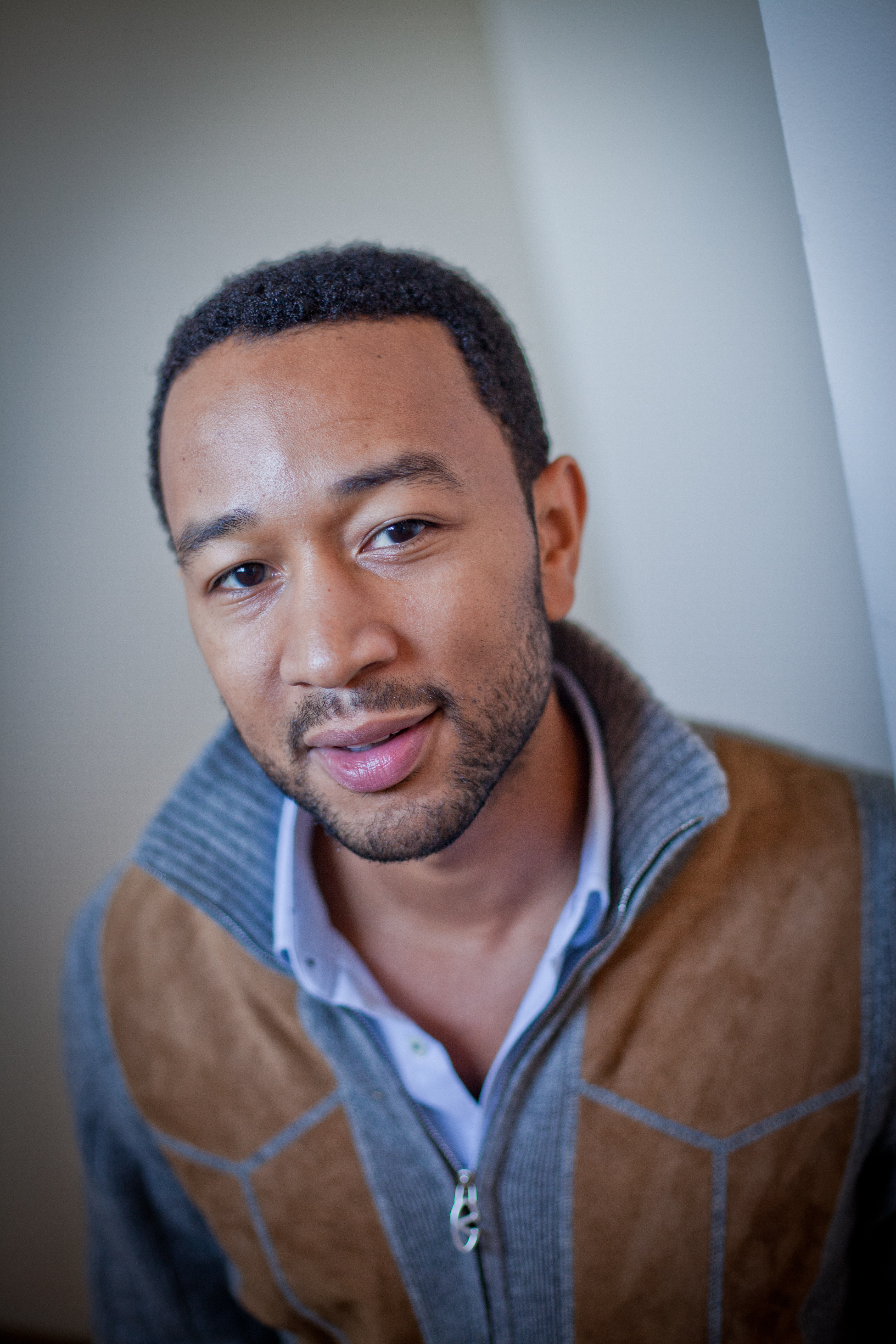This is a detailed image of the singer John Legend. He is smiling and appears content. John has short, slightly curly hair and a mustache-beard combo. He is dressed in a gray zip-up jacket with brown vertical stripes and some leather detailing on the front, with the collar stylishly popped up. Underneath the jacket, he wears a light blue collared button-down shirt, with the top two buttons open. The photo crops up to his chest, and he stands against a simple, plain white background.